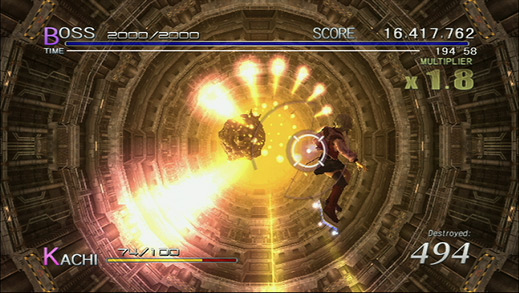In this detailed screenshot from a video game, we observe a dynamic scene unfolding within a large, cylindrical structure characterized by tan and brown hues. The central focal point is a bright yellow light emanating from the bottom of the cylinder. A formidable, brown, circular, monstrous creature is situated there, launching orange orbs of light upward. The character, a girl wearing a red, black, and pink outfit, navigates this perilous environment on a futuristic hoverboard, which emits a blue glow. 

At the top of the screen, game statistics are prominently displayed: "Boss 2000/2000," a score of "16,417,762," "Multiplayer x 1.8," and "Destroyed 494." Positioned in the bottom left corner is the name "Kachi (K-A-C-H-I) 74/100." The vivid description and the numeric displays suggest an intense, high-stakes part of the game, possibly a boss fight, underscored by the chaotic blend of fire, explosions, and hovering mechanics.